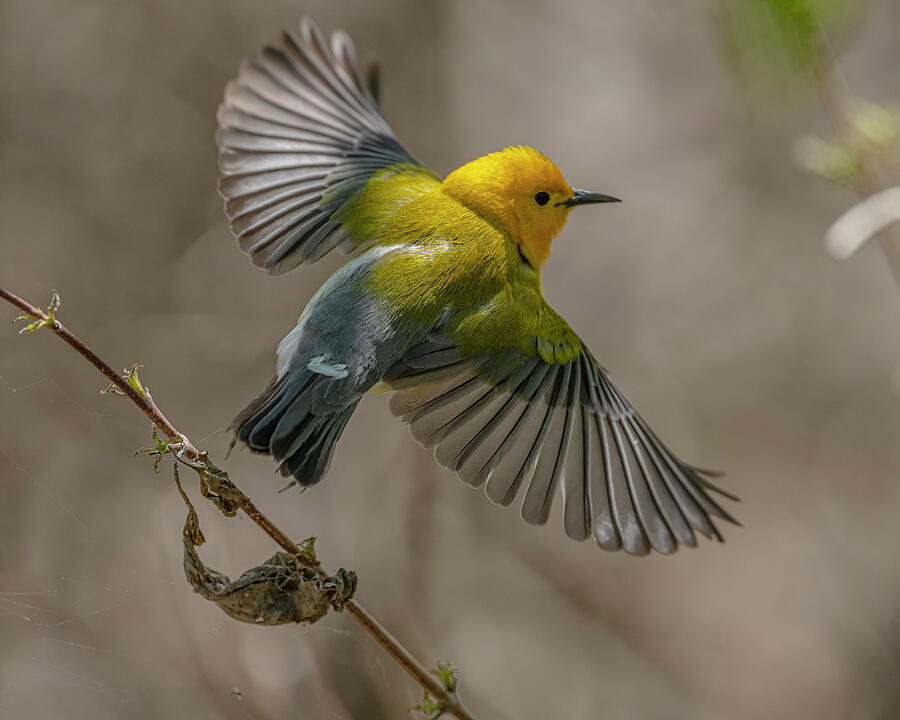In this crisp, clear photograph, the central focus is a stunning bird captured in exquisite detail. The bird's wings are fanned out, displaying feathers so well-defined you can see each one distinctly. Its tail feathers are a mix of darker and lighter shades of gray, and there are subtle off-white markings as well. The bird's head and the upper portion of its back are adorned with a striking gold color, blending into a beautiful olive green around its body. The bird's eyes are a deep black, and it has a sleek black beak. The delicate, light gray feathers of its wings add to its graceful appearance.

Behind the bird's tail, there is a slender tree branch with a coarse brown texture, adorned with a mix of gray and tan leaves, and a hint of green peeking through. The background features a blend of brown and white shadowing, with a splash of green from another leaf, creating a natural, serene setting that complements the bird’s radiant plumage.